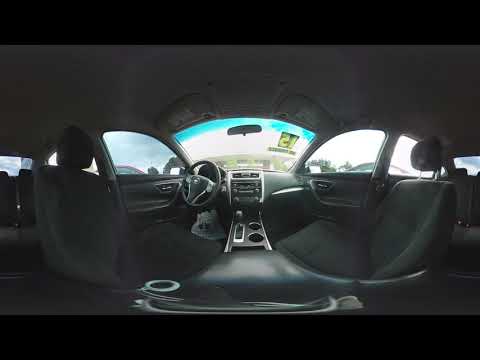This panoramic photograph, taken from the middle back seat of a car, showcases the impeccably detailed interior. The shot captures the black leather front seats—both the driver and passenger seats—positioned around a central console. The console houses an automatic gear shifter, two cup holders, and a modern radio unit, all framed by dark gray and silver trim. The dashboard is visibly adorned with a "15" sticker on the passenger side, indicating the model year of the vehicle. The steering wheel, colored in a matching dark gray, is prominent on the left, adjacent to the driver's side window. Through the car windows, the bright blue sky and the hoods of other cars can be faintly seen. The panoramic effect slightly curves the perspective, giving an encompassing view of this sleek, meticulously maintained automobile.